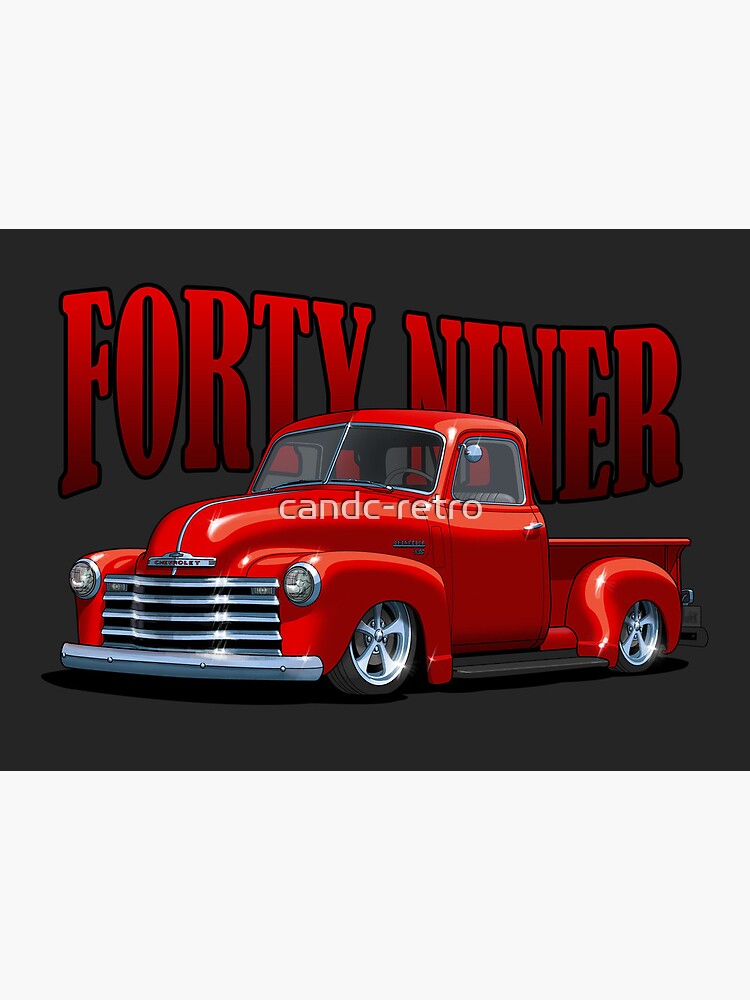The image features a stylized, computer-generated depiction of a cherry red, vintage pickup truck, likely from the 1950s or 60s. This two-door truck, facing left and slightly frontward, has a prominent horizontal silver grille, chrome door handles, and silver wheels. It also sports a short bed at the back. The truck is set against a black background. Prominently displayed above and partially behind the truck in bold red capital letters is the word "49ER." The letters "N" "I" and "N" from "Niner" slightly overlay the truck's windshield, with pieces visible through the glass. Just beneath the windshield, the truck has the white inscription "CAN DC RETRO" in a stylized font. The overall aesthetic combines cartoon-like and vintage elements, emphasizing a nostalgic, retro feel.